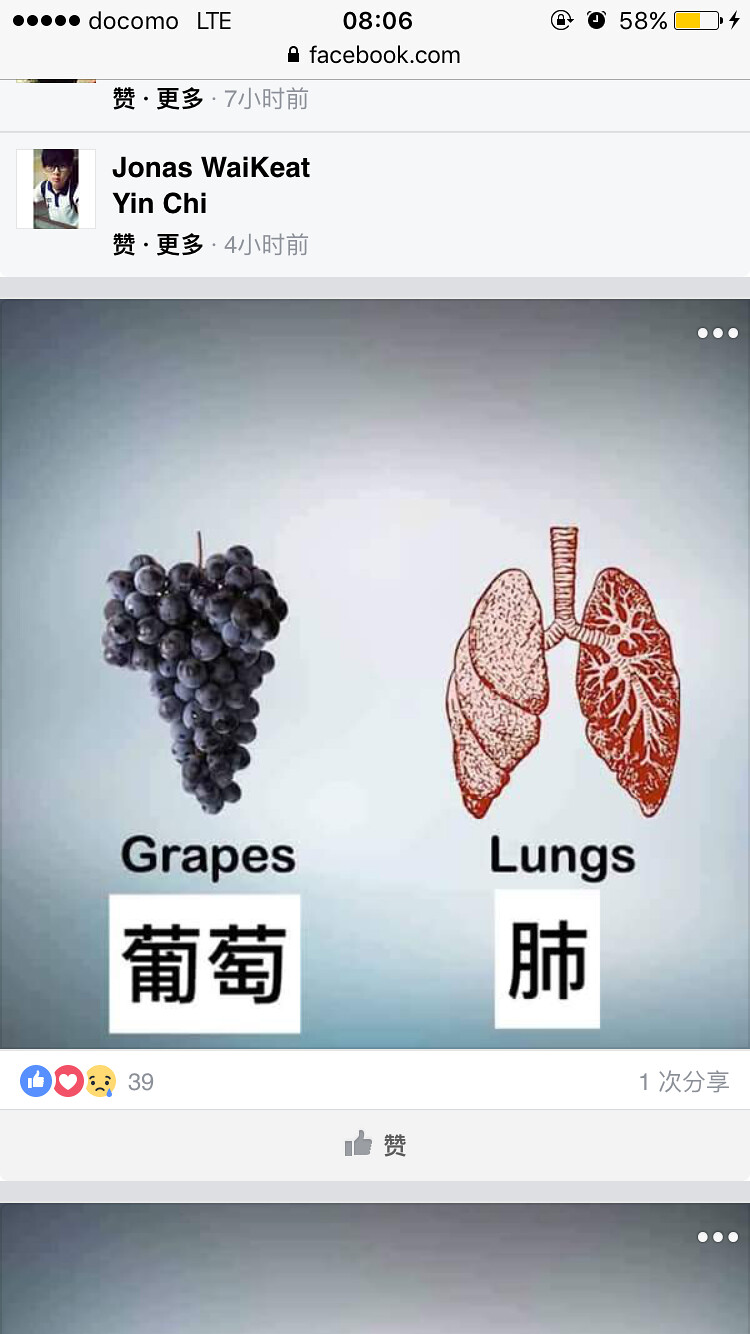This screenshot captures the front of a mobile phone displaying a Facebook page. At the top, the notification bar reads "DOCOMO LTE" on the left, displays the time as 08:06 under "Facebook.com" in the middle, and shows that the battery percentage is at 58% on the right. Below this, the Facebook post is authored by Jonas Vaughn, Yen-Chi, followed by Chinese or Japanese characters. The post features an image with two parts: on the left, a cluster of purple grapes labeled "grapes" with additional Chinese text, and on the right, a depiction of red lungs labeled "lungs" also accompanied by Chinese text. The layout draws a comparison between the shape of the grapes and the lungs. At the bottom of the post, there are interaction icons, including a thumbs-up emoji and the number 39, as well as three dots in a gray bar. Another partially visible post is shown beneath this one.